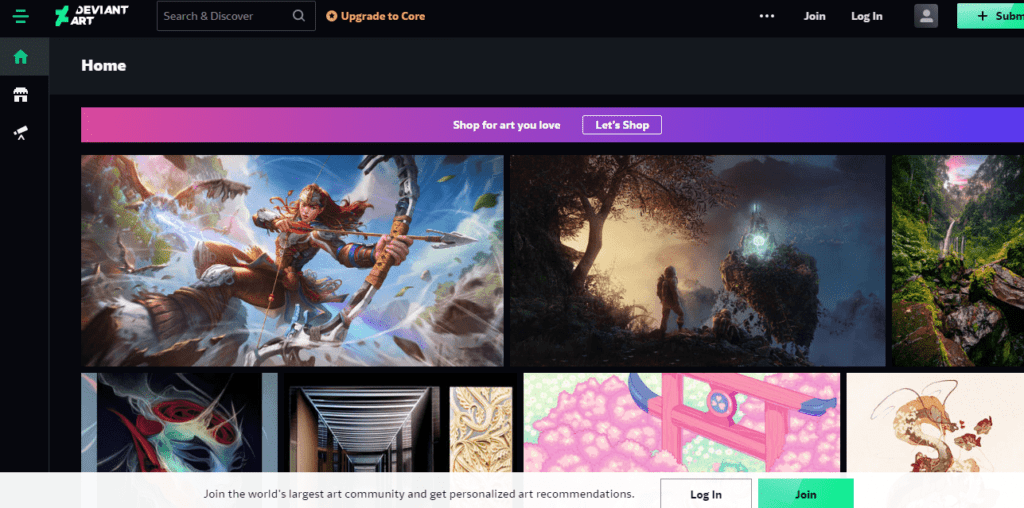This image is a screenshot of the DeviantArt website. At the top, the word "DeviantArt" is displayed in white font alongside a green logo. Directly below this is a grey search box labeled "Search and Discover." In yellow text, there's an upgrade option titled "Upgrade to Core," featuring a black star in the center of a yellow circle. To the right, there are buttons labeled "Join," "Log In," and a partially visible "Submit" button.

On the left side, the navigation bar includes a home icon followed by two additional icons—a house and a telescope. Prominently displayed in large white letters on a black background is the word "Home." Below, a banner reads "Shop for Art You Love" with a prompt, "Let's Shop."

The main section features various digital images and photographs. One image depicts a woman with long red hair wielding a bow and arrow. Another showcases a person standing and gazing at a glowing light in a forest setting, featuring a prominent tree. Additional images include a dragon in the bottom right corner and a Japanese torii gate.

Underneath these images, a text banner invites viewers to "Join the world's largest art community" and promises personalized art recommendations. This is followed by "Log In" and "Join" buttons for user engagement.